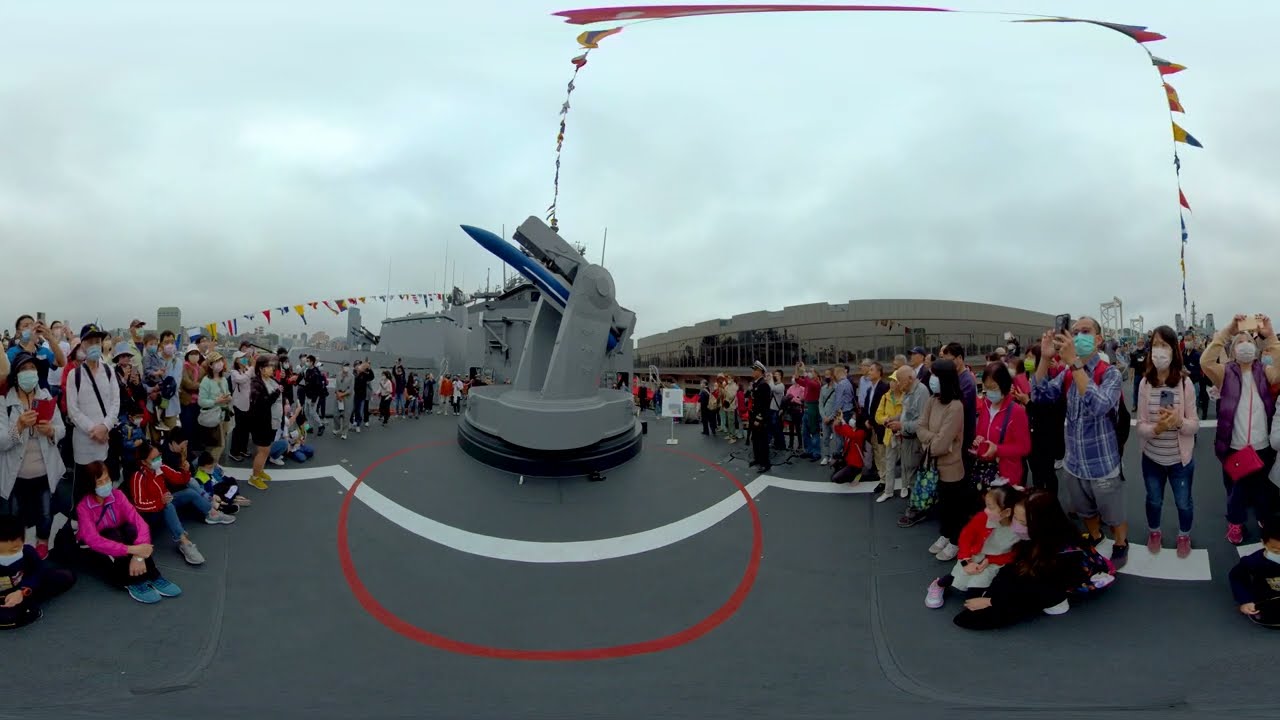In the panoramic 360-degree image of an outdoor scene, a group of people stands on gray pavement marked with white and red lines, encircling a large blue missile-like device on a rotating pedestal. This apparatus, which looks like a missile launcher, is capable of altering the projectile's elevation and orientation via horizontal and vertical axes. Many of the spectators, some clad in military uniforms and nearly all wearing face masks, are capturing the scene with their phones. The event appears to be a formal presentation, with flags hanging above and around the audience. The setting is adjacent to a long, gray institutional-style building with extensive glass walls. Overhead, the overcast sky adds a pale blue-gray backdrop to the scene, filled with textured clouds.